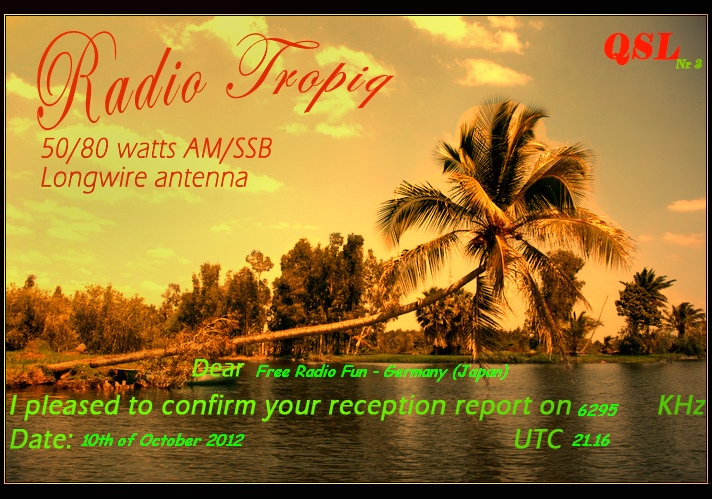The image appears to be a vintage-style postcard or a screenshot of a PowerPoint slide with a sepia-toned filter, evoking a late afternoon or sunset atmosphere. The background depicts a tranquil tropical scene, with a large palm tree leaning over a serene body of water, flanked by other trees. The partly cloudy sky and hues of yellow, brown, gray, and a hint of dark green further enhance the nostalgic feel.

In the upper left corner, in red cursive text, it reads "Radio Tropic," followed by "50-80 watts AM-SSB long wire antenna" in a smaller, regular font. On the upper right corner, bold and also in red, it says "QSL NR3." At the bottom of the image, in green text, it states, "Dear Free Radio Fund Germany (Japan), I am pleased to confirm your reception report on 6295 kHz, date 10th of October 2012, UTC 2116." This text suggests a formal acknowledgment of a radio signal reception between two parties, possibly as part of a radio hobby or communication verification process.